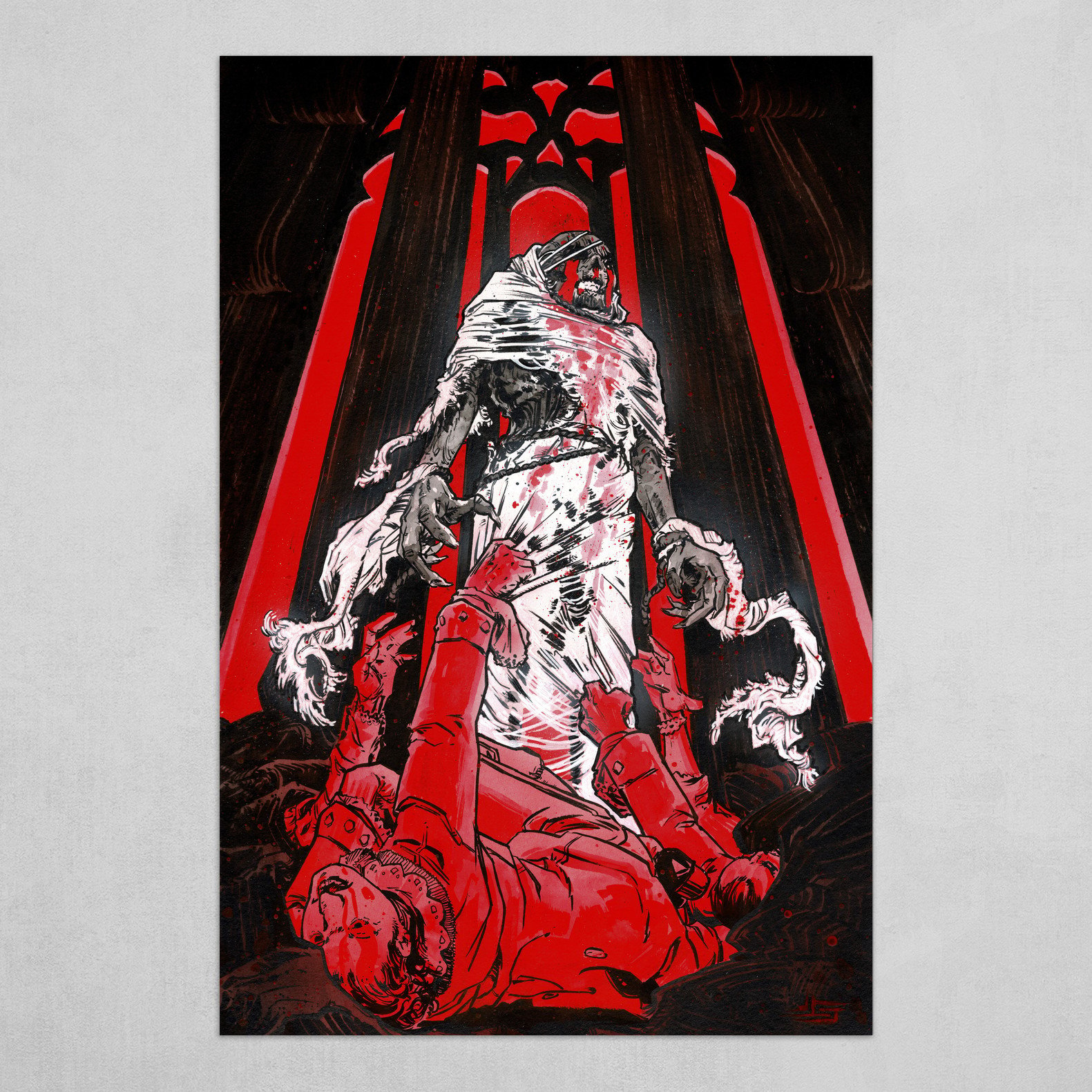The image is a detailed, ominous cartoon-style painting dominated by red, black, white, and touches of gray. Centered within the composition is a sinister skeletal figure draped in a tattered white robe stained with red splatters, giving the appearance of blood. This eerie figure, resembling a demonic creature, stands imposingly above a prone man in the foreground. The man, garbed entirely in red and sporting a fancy collar, lies on his back with his mouth agape and his head thrown back, frantically clutching at the figure's shredded robe. His red body and face, from which red liquid appears to be dripping, emphasize a scene of despair and struggle. Surrounding this central drama, the backdrop features towering black columns and a large, foreboding doorway. Red light pours through the window, casting an eerie, blood-like glow over the entire scene, enhancing the painting's sense of dread and horror.